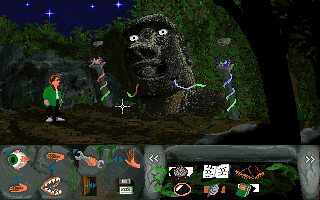This image depicts a scene from a side-scrolling video game. The main character, who is facing to the left, is dressed in a green coat over a white shirt, paired with black pants and white shoes. The character has brownish hair and appears to be looking off into the distance. In the background, there's a striking stone figure with wide-open eyes, reminiscent of an Easter Island statue, gazing upwards.

Prominently featured on the screen are crosshairs, suggesting a targeting or focus mechanic in the game. At the bottom of the screen, a HUD (Heads-Up Display) showcases various icons, possibly representing different game functions or items. These icons include a tooth, an eyeball, a wrench, and a hand. Nearby, another section displays additional symbols that resemble a map, sunglasses, a rock, a leaf, a spear, and a book, hinting at the diverse elements and interactive objects within the game.